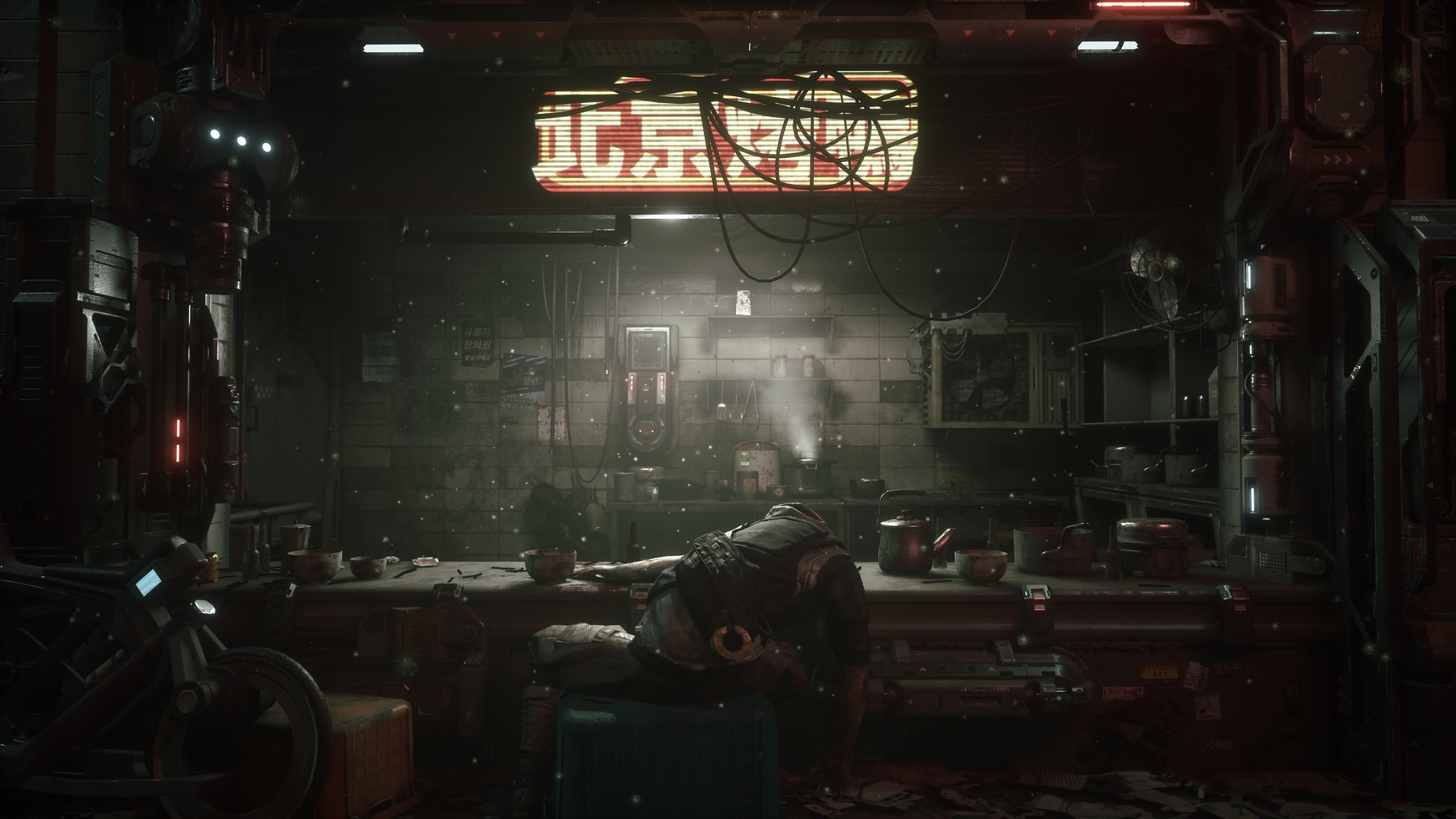The image depicts a dark, industrial-style kitchen or restaurant scene, possibly a still from a movie. The back wall, constructed of large gray bricks, features an assortment of cooking utensils such as pots and pans hanging from it, with additional shelves stocked with various items on both the back and side walls. A stove is situated against the back wall, emitting steam from a pot, indicating active cooking. In the foreground, there is a long counter or bar with multiple items including bowls, spoons, pots, a teapot, and a bonsai tree. In front of the counter, a large, obese person appears slumped over on a green bench, with their head and arm resting on the table as if they are passed out. The lighting is minimal and primarily concentrated near the back wall, creating a dark atmosphere. Overhead, a red neon sign with white Chinese writing, partially obstructed by an electrical cord, reads "Beijing Congee and Noodles." The overall scene evokes a sense of a futuristic, possibly dystopian environment.